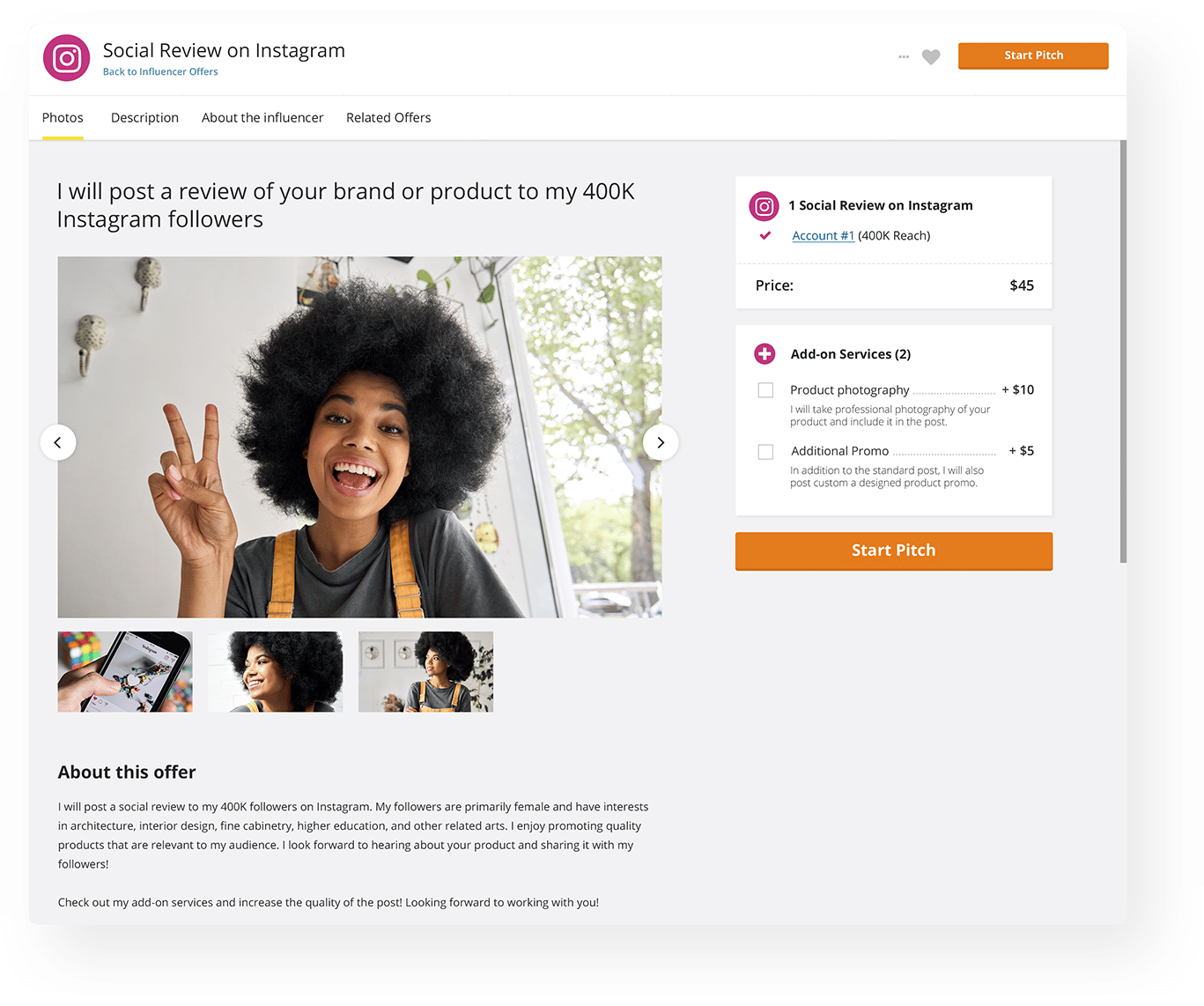This is a detailed caption for someone describing a website screenshot:

"This screenshot showcases a webpage focused on influencer marketing through Instagram. In the top left corner, the Instagram logo is prominently displayed alongside the title 'Social Review on Instagram.' On the top right corner, there is an eye-catching orange bar labeled 'Start Pitch,' accompanied by a grayed-out heart icon.

Just below this header, a row of four clickable links includes 'Photos,' 'Description About the Influencer,' and 'Related Offers.' An engaging statement follows, reading, 'I will post a review of your brand or product to my 400,000 Instagram followers,' alongside a photograph of a woman flashing a peace sign.

Beneath this central image are three thumbnail photos. The left thumbnail shows a person holding a cell phone, while the middle and right thumbnails feature the same woman from the main image. On the right side of the screen, there's informative text detailing the influencer's reach—'Social Review on Instagram. Account number: 400,000 reach.' The price for the service is indicated at $45.

Further down, a menu lists add-on services, with two options: 'Product Photography' for an additional $10 and 'Additional Promo' for $5. At the very bottom, a section titled 'About This Offer' contains a paragraph of text, though the text is too small to be read clearly in this screenshot."